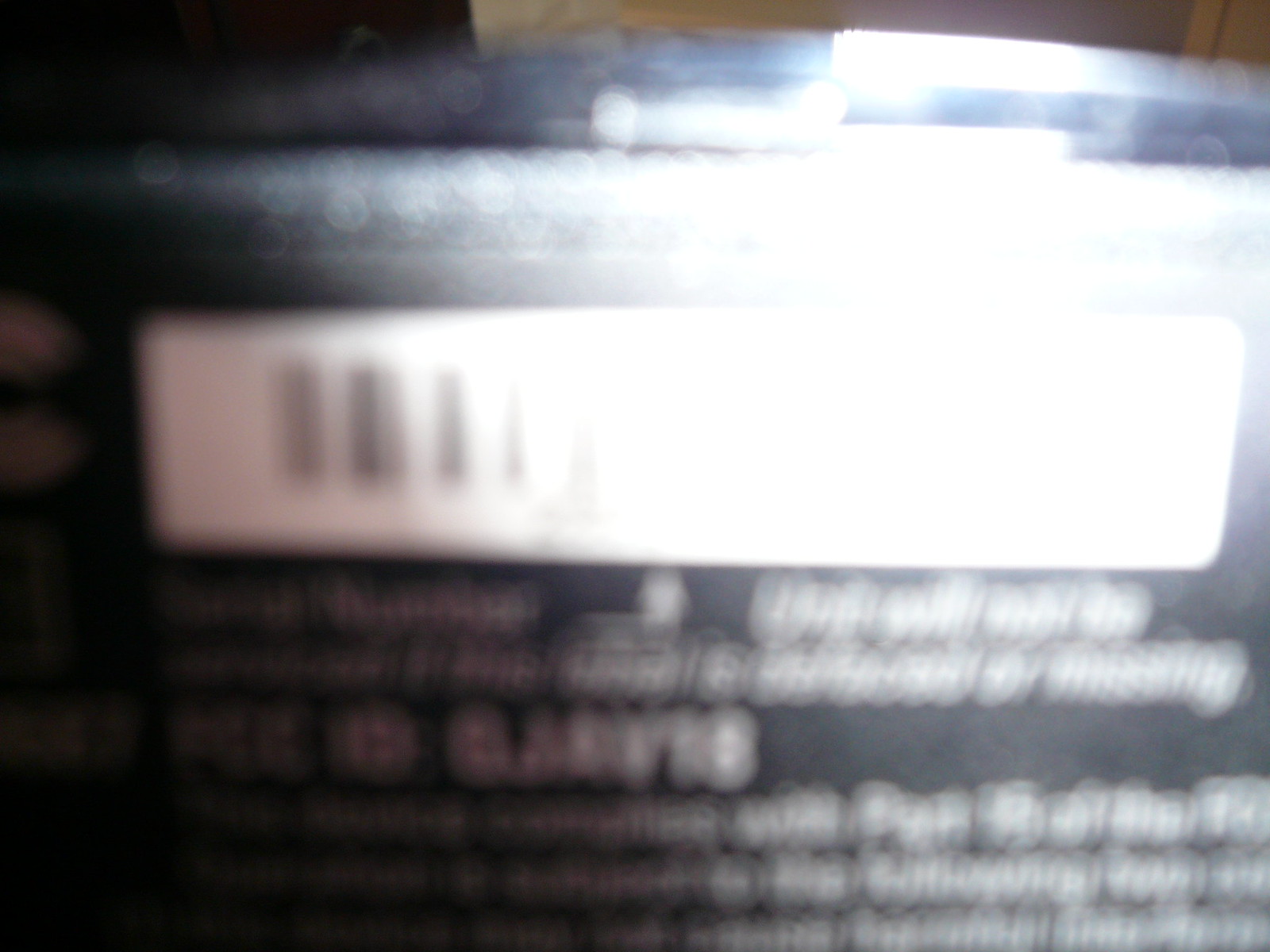This photograph captures a close-up, horizontal shot of a can. The image is notably blurred, obscuring finer details and edges. The can appears to be of a flat, possibly rectangular type, though the blurriness makes it difficult to confirm its exact shape or dimensions. Prominently featured in the image is a white label located just above the center of the can, displaying a barcode on its left end. The background behind the can is a dark bluish-gray with indistinct white lettering, contributing to the overall mystery and texture of the scene.